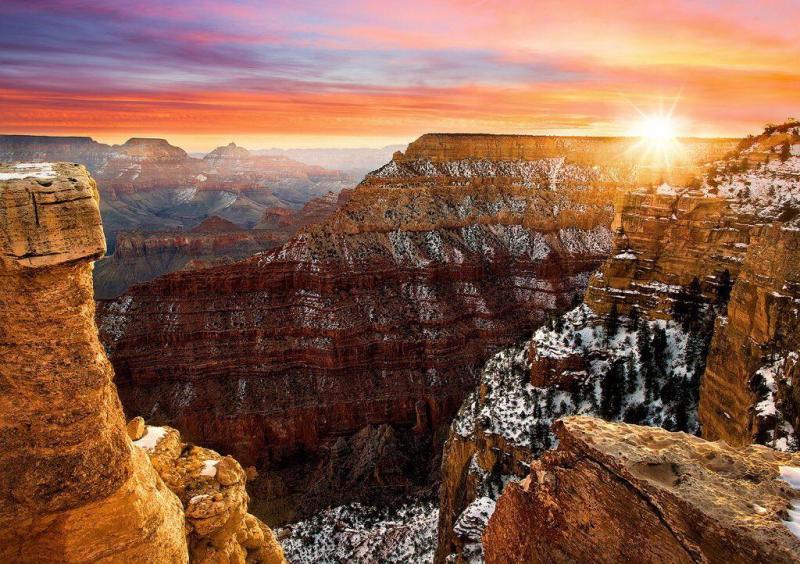This highly edited and visually synthetic photograph captures an expansive and jagged cliff and canyon landscape, reminiscent of the Grand Canyon in winter. The cliffs, composed of gray and tan stone, stretch as far as the eye can see, interspersed with patches of ice and clusters of pine trees along with other stunted vegetation. The sky is a vibrant, otherworldly mix of orange, blue, and purple hues, with an orange sun rising on the top right of the image. The sun's rays illuminate some of the rocks, highlighting their rugged and jagged nature. The overall scene is surreal, with mismatched shadows creating an ethereal atmosphere. The rectangular image, with the longer sides running horizontally, emphasizes the panoramic scope of this dramatic landscape.